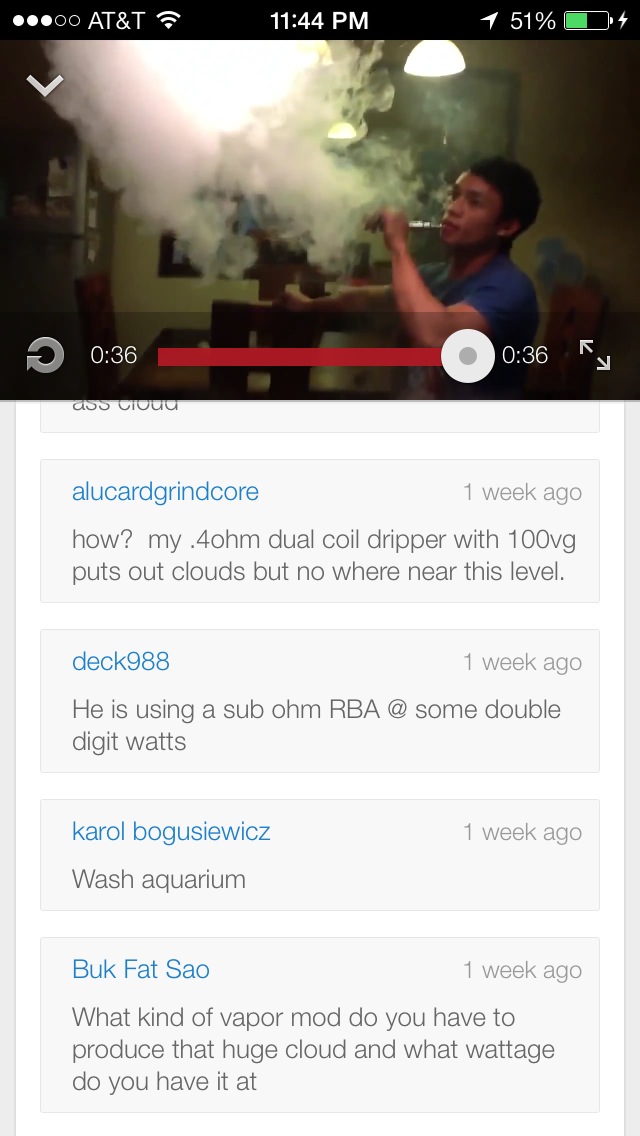The image is a detailed screenshot taken from a mobile device displaying a YouTube video interface. At the top of the screen, it indicates the user is on an AT&T network with 51% battery life and the time is 11:44 PM. The main content is a 36-second video paused at the very end, showing a young Asian man in a light blue shirt vaping, with smoke filling the room around him. His arm is raised towards his mouth as he exhales a large cloud of vapor. Underneath the video, several comments are visible, including one from a user discussing vape equipment, mentioning a .4 ohm dual coil dripper with 100% VG and comparing it to the vaper's large clouds. The overall colors in the screenshot include black, white, green, red, tan, and light blue, and the interface elements such as the minimize/maximize icons are present on the screen.